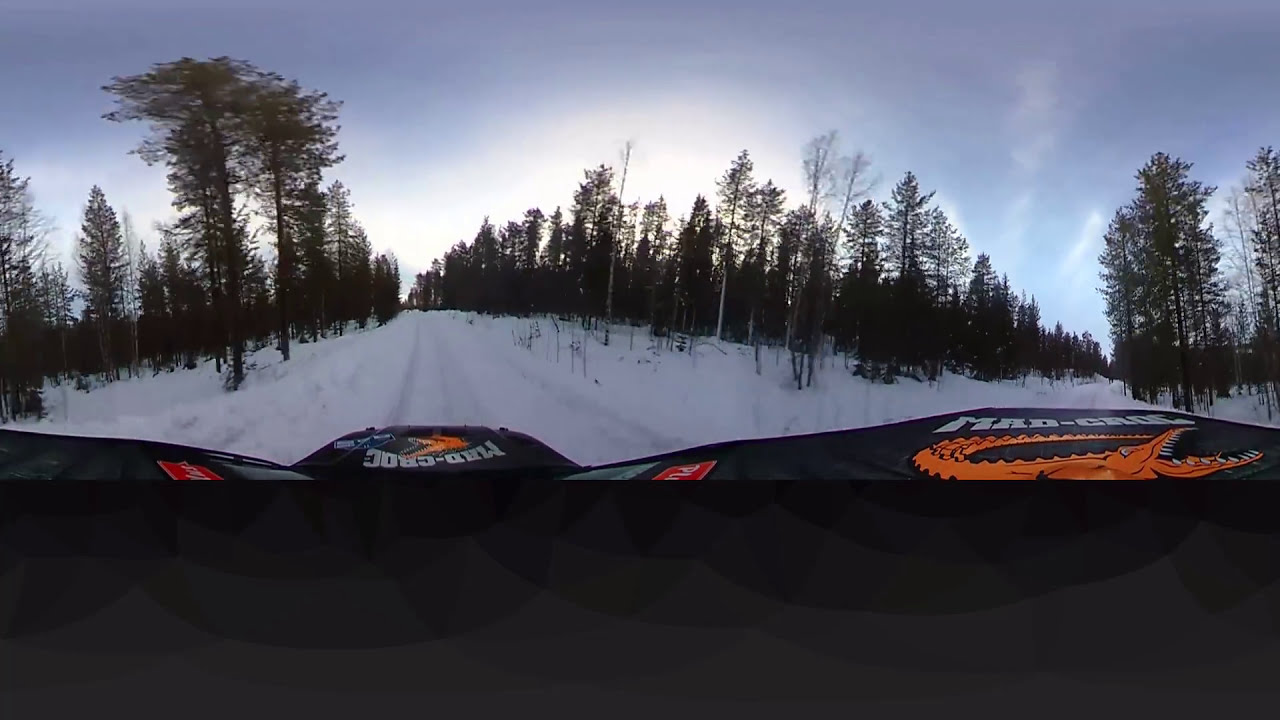A person is riding a black snowmobile along a snowy path surrounded by thin trees with greenish leaves. The snowmobile's black hood dips down and then slightly peaks back up in the middle. Prominently displayed on the front are two identical stickers featuring an orange crocodile with its mouth open, labeled "MAD-CROC." One sticker is placed normally, while the other is flipped upside down. There are additional red and green tags on the snowmobile, but they are too small to read clearly. The snow on the path looks freshly fallen and hard-packed, with visible tracks indicating recent travel. The scene is bright, with a mix of pine trees and leafless deciduous trees, creating a wintry backdrop.